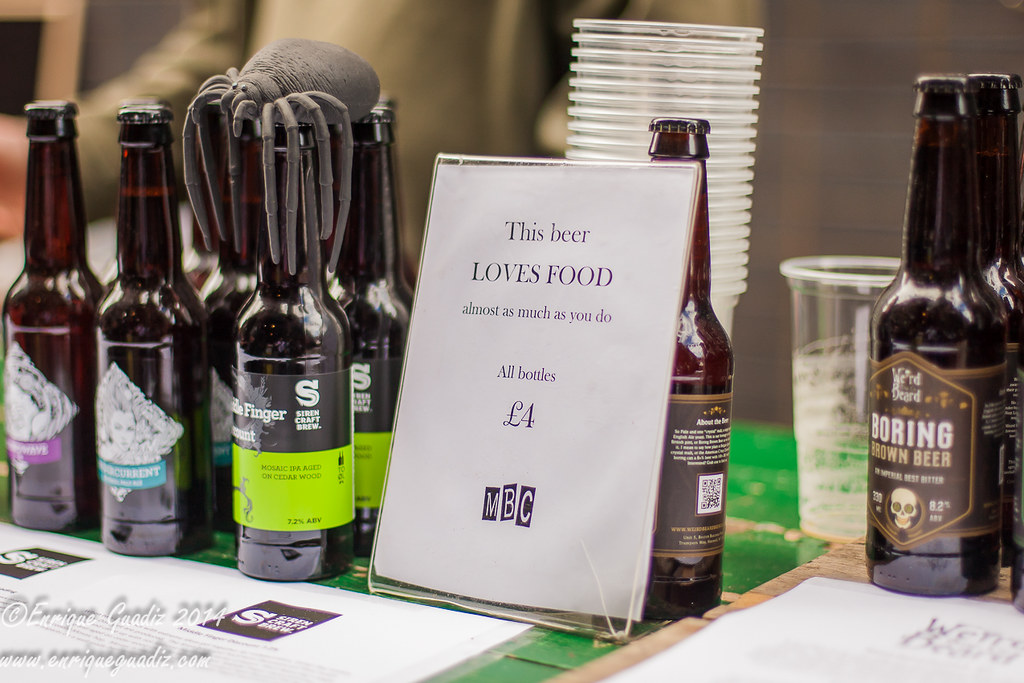This detailed photograph captures an inviting scene centered around a green-painted wooden table adorned with numerous brown beer bottles. Dominating the composition is a prominent white sign leaning against one of the bottles. In black text, the sign humorously declares, "This beer loves food almost as much as you do. All bottles, $4, MBC," where "MBC" appears in white text within brown boxes, though its meaning remains unclear. To the left, six bottles are arranged, one intriguingly topped with a large toy spider. Behind one of these bottles, several plastic cups are stacked, ready for use. The background reveals more beer bottles, enhancing the convivial and promotional atmosphere.